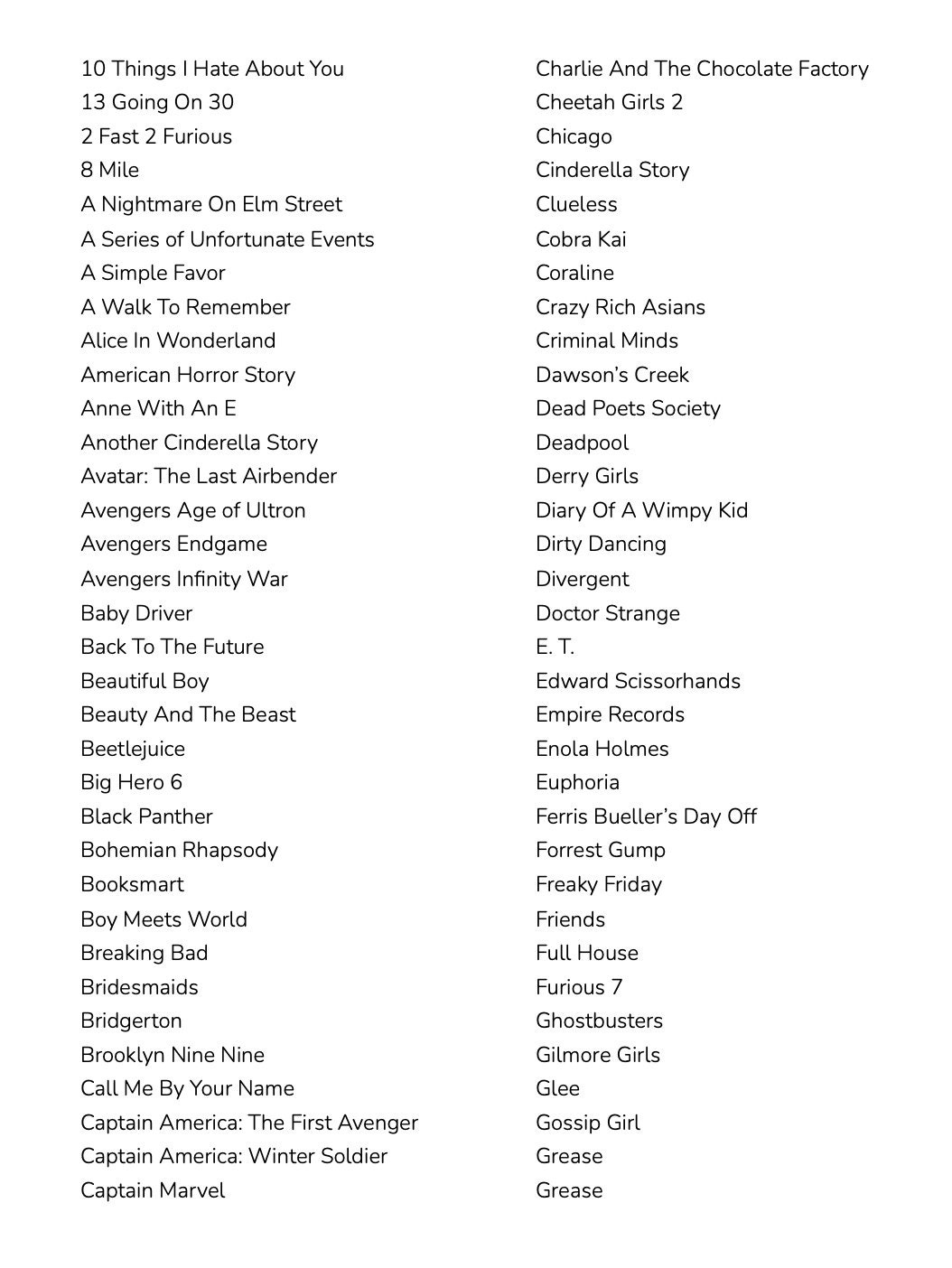Screenshot of a list of movies and TV shows in alphabetical order:

A comprehensive and varied alphabetical list showcasing a diverse collection of movies and TV shows. This detailed screenshot includes:

- **"10 Things I Hate About You"**
- **"13 Going on 30"**
- **"2 Fast 2 Furious"**
- **"8 Mile"**
- **"A Nightmare on Elm Street"**
- **"A Series of Unfortunate Events"**
- **"A Simple Favor"**
- **"A Walk to Remember"**
- **"Alice in Wonderland"**
- **"American Horror Story"** (TV show)
- **"Anne with an E"** (TV show)
- **"Another Cinderella Story"**
- **"Avatar: The Last Airbender"** (TV show)
- **"Avengers: Age of Ultron"**
- **"Avengers: Endgame"**
- **"Avengers: Infinity War"**
- **"Baby Driver"**
- **"Back to the Future"**
- **"Beauty and the Beast"**
- **"Beetlejuice"**
- **"Big Hero 6"**
- **"Black Panther"**
- **"Bohemian Rhapsody"**
- **"Booksmart"**
- **"Boy Meets World"** (TV show)
- **"Breaking Bad"** (TV show)
- **"Bridesmaids"**
- **"Bridgerton"** (TV show)
- **"Brooklyn Nine-Nine"** (TV show)
- **"Call Me By Your Name"**
- **"Captain America: The First Avenger"**
- **"Captain America: The Winter Soldier"**
- **"Captain Marvel"**
- **"Charlie and the Chocolate Factory"**
- **"The Cheetah Girls 2"**
- **"Chicago"**
- **"A Cinderella Story"**
- **"Clueless"**
- **"Cobra Kai"** (TV show)
- **"Coraline"**
- **"Crazy Rich Asians"**
- **"Criminal Minds"** (TV show)
- **"Dawson's Creek"** (TV show)
- **"Dead Poets Society"**
- **"Deadpool"**
- **"Derry Girls"** (TV show)
- **"Diary of a Wimpy Kid"**
- **"Dirty Dancing"**
- **"Divergent"**
- **"Doctor Strange"**
- **"E.T. the Extra-Terrestrial"**
- **"Edward Scissorhands"**
- **"Empire Records"**
- **"Enola Holmes"**

Note: This list includes both movies and TV shows, exhibiting a broad spectrum of genres and time periods.